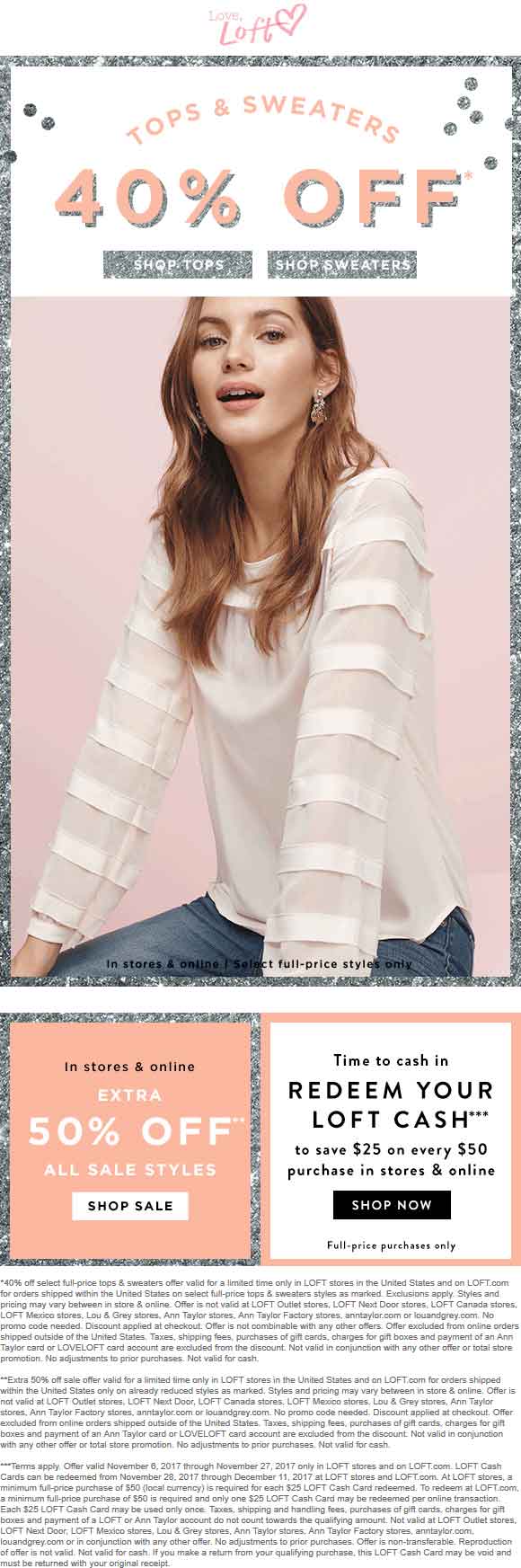The image is a vertical advertisement from Love Loft, likely designed for email distribution, websites, or smart devices. It features a young woman directly facing the camera, wearing a top, and appears on a white background displayed on a computer screen. The ad has a whitish-gray border surrounding it.

At the top, a small heart icon and the "Love Loft" brand name are displayed. The central section of the image announces a promotional offer: "Tops and Sweaters 40% Off" in white letters against a peach-colored background. Further details indicate that the sale applies to select full-price styles, available in stores and online, with an additional 50% off all sale styles.

Below this, additional promotional information is set against a white background framed by a peach border. It reads: "Time to Cash In," inviting customers to redeem their Loft Cash to save $25 on every $50 purchase, applicable in stores and online. A black rectangular button marked "Shop Now" in white letters encourages immediate action, with a note indicating the offer is for full-price purchases only. The advertisement concludes with three paragraphs of fine print at the bottom.